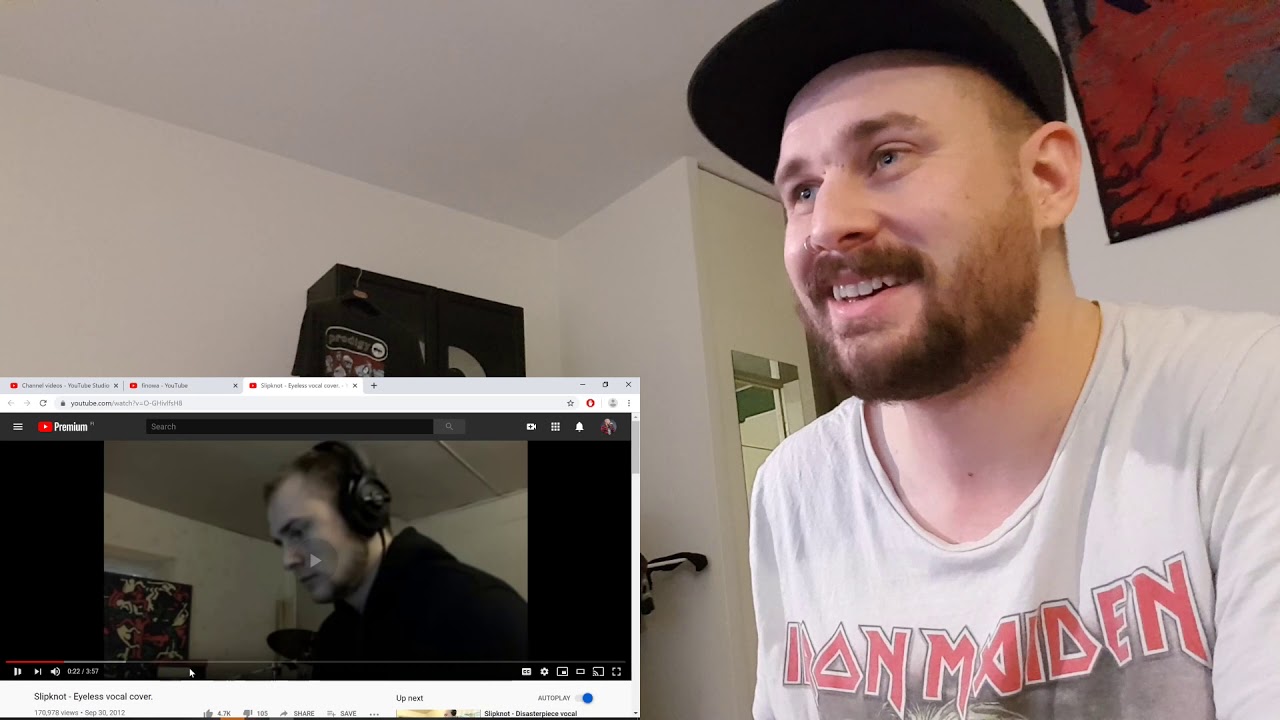In the image, a man with a light brown beard and a nose ring in his right nostril is watching a YouTube video, displayed in the bottom left corner of a browser window. He has light-colored eyes, possibly blue or gray, and is wearing a white shirt with the name "Iron Maiden" written in red across the chest. At the top right of the image is a white wall adorned with a red painting, although the painting's details are unclear. To the middle left, a black shirt with a white and red logo is hanging on a closet door in the background. The browser window at the bottom left shows three open YouTube tabs; the active tab features a video thumbnail of a man wearing black headphones and a black sweater, and the video title appears to be "Slipknot Eyelash Vocal Power." Additionally, an ad block icon, characterized by a red circle with a white logo, is visible at the top right of the browser.